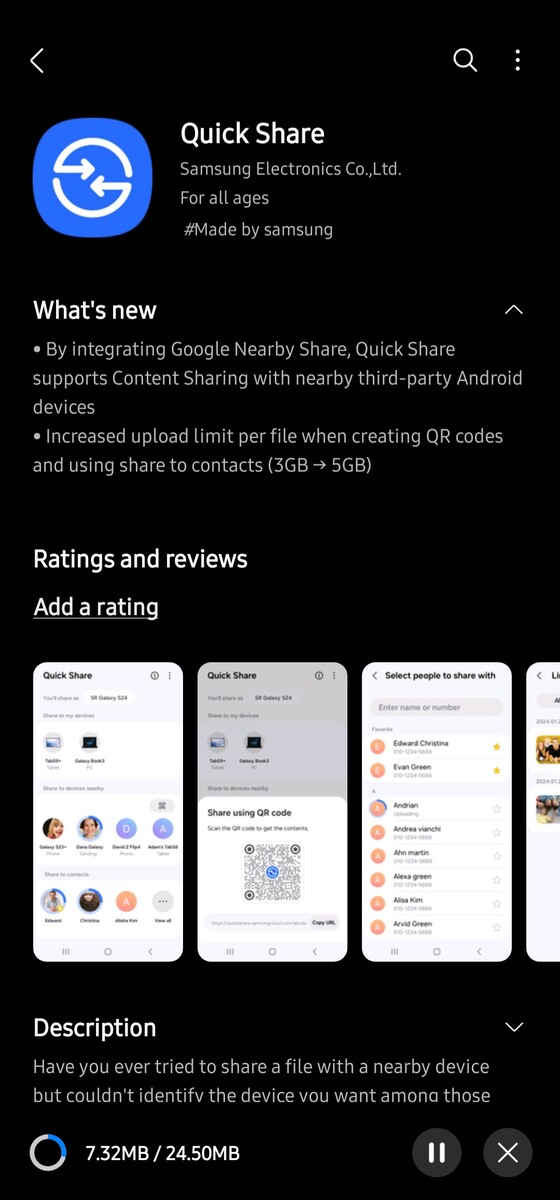In the screenshot, we see a section of an app interface. Starting in the upper left corner, there's a blue square with rounded corners. To its right, in white text, it reads, "Quickshare Samsung Electronics Company Limited for all ages #madebySamsung." Below this header, there's a "What's new?" section:

- A bullet point states, "By integrating Google Nearby Share, Quickshare supports content sharing with nearby third-party Android devices."
- Another bullet point mentions, "Increased upload limit per file when creating QR codes and using share to contacts from 3 gigabytes to 5 gigabytes."

Further down, in bold white text, it says, "Ratings and Reviews," followed by an option to "Add a rating." This section displays images of screenshots. Beneath the images, in white text, there's a "Description" section, which starts with the question, "Have you ever tried to share a file with a nearby device but couldn't identify the device you want among those?"